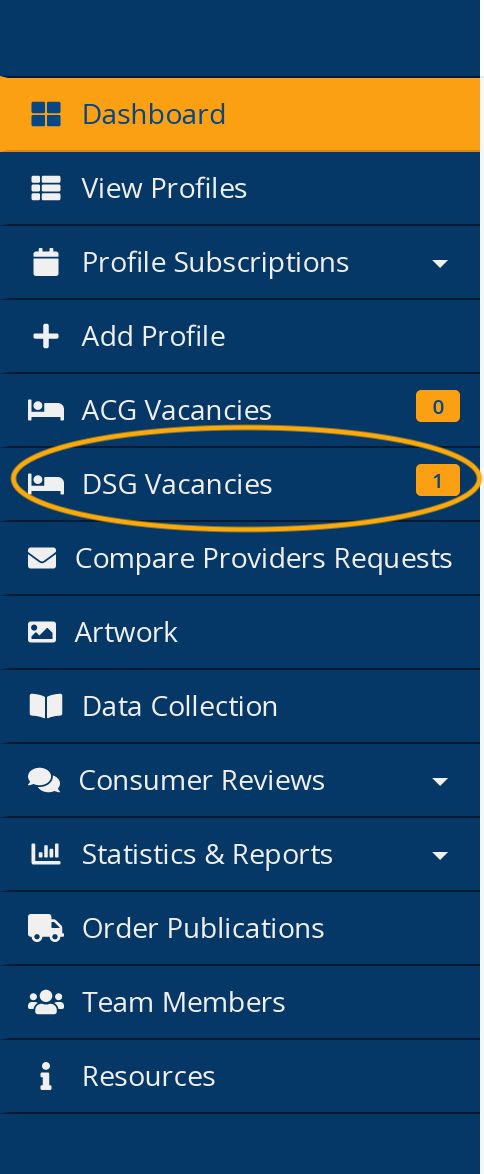This is a detailed color image depicting a section of a web page interface. The background is predominantly dark blue with contrasting white text. Toward the top of the image, an orange band spans the width of the page, featuring blue text. Above this orange band and occupying the uppermost part of the image is a blank blue row, free of any text or icons.

Below this blank row is the orange-yellow band which is on the second row. In the orange-yellow band, the word "Dashboard" is prominently displayed in blue text, accompanied by an icon depicting a window. 

The interface is structured into several sections, each separated by thin black lines. Down the left side of the page, a vertical strip features various icons. Immediately following the "Dashboard" section, there are clickable menu items including "View Profiles," "Profile Subscriptions" marked with a downward arrow, and "Add Profile."

Further down the list, the section titled "ACG Vacancies" shows the number 0 inside an orange square, while "DSG Vacancies" displays the number 1 in an orange square. This particular "DSG Vacancies" section is highlighted with a yellow oval around it.

Additional menu options include "Compare Providers' Requests," "Artwork," "Data Collection," "Consumer Reviews," "Statistics and Reports," "Order Publications," "Team Members," and "Resources."

The mention of consumer reviews, statistics, and reports suggests this interface is likely part of a back-end application for a consumer-focused website or application. The presence of the "ACG Vacancies" and "DSG Vacancies" icons, which resemble beds, hints that the application might be related to travel services where vacancies and consumer profiles are managed, though this remains speculative.